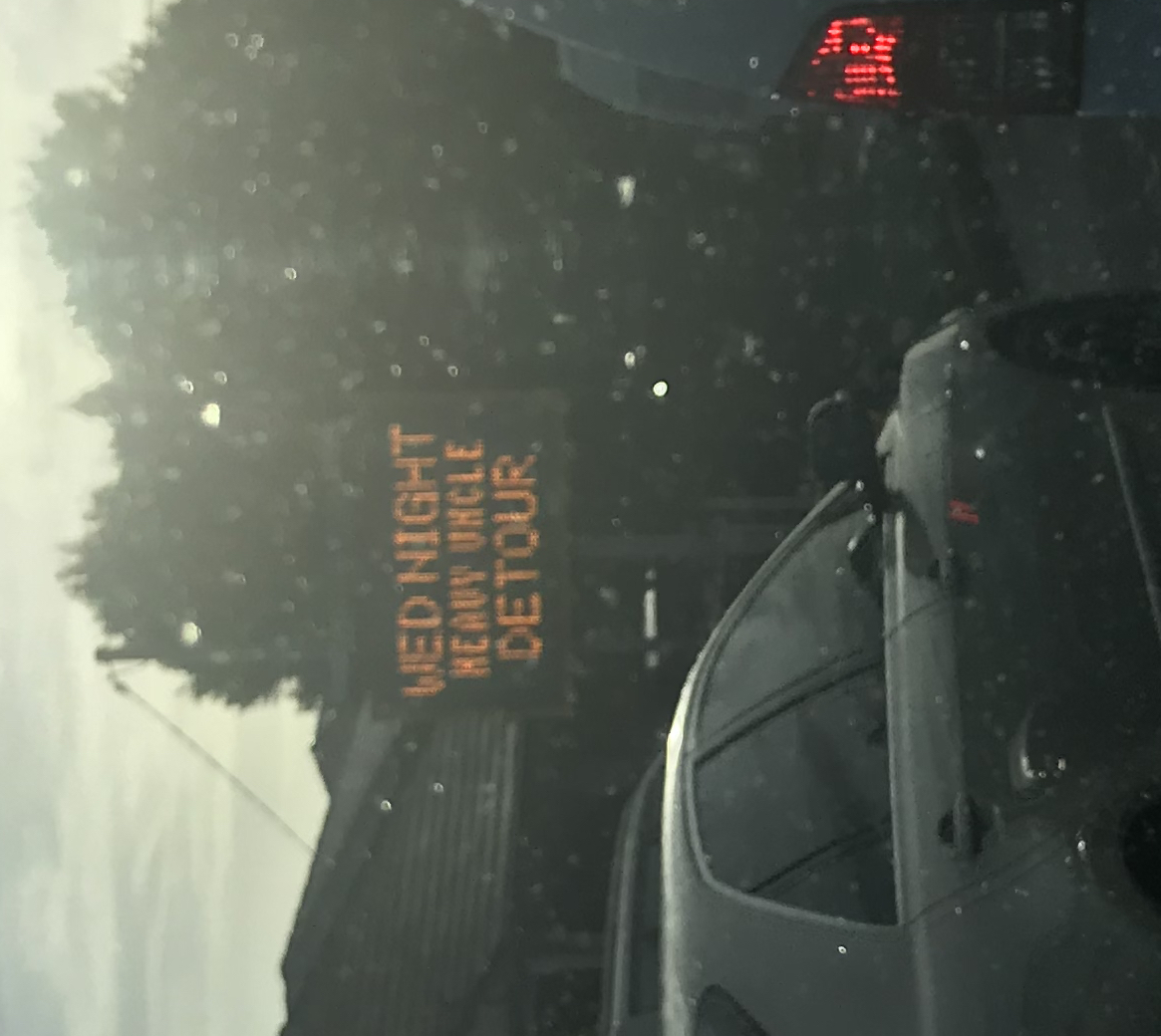This photograph, which appears to be rotated 90 degrees counterclockwise, depicts a scene taken through a dirty windshield or lens. In the bottom left corner, there is a gray sedan. Prominently displayed is a traffic sign with black and orange text that reads, "Wednesday Night Heavy Vehicle Detour," although the text might initially appear confusing. In the background, there are several trees and the rooftops of some houses. The sky is gray and cloudy, suggesting the photo was taken at dusk. There is noticeable heavy traffic in the area, and the overall atmosphere is quite dark and subdued.